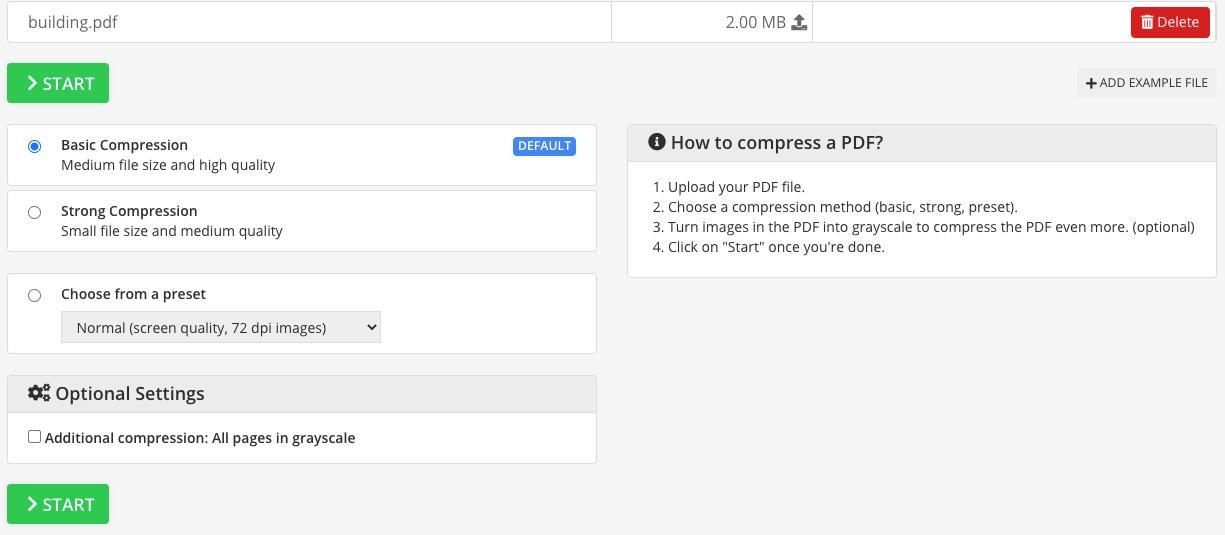The image displays a user interface for a document compression tool. 

In the upper left-hand corner, the filename "building.pdf" is displayed in lowercase letters. To the right, it shows the file size as "2.00 MB" alongside an icon of a hard drive with an arrow pointing upwards, indicating an upload. 

In the upper right-hand corner, within a red rectangular box, there is an icon of a trash can and the word "DELETE" to its right.

On the main web page, in the upper left-hand corner, is a rectangular box with the word "START" in uppercase, followed by a greater-than symbol (>). To the far right, there is another rectangular box shaded gray with a plus sign and the label "ADD EXAMPLE FILE" in uppercase letters.

On the left-hand side of the main interface, there are several options available:
1. The first option, which is circled, is labeled "Basic Compression" and includes the settings: Medium file size and High quality (default).
2. The next option reads "Strong Compression" and includes settings for a small file size and medium quality.
3. The final option is "Choose From a Preset," which features a drop-down menu with the preset set to "Normal screen quality, 72 dpi images."

Below these options, there is a checkbox labeled "Optimal Settings" for users who prefer additional compressions and converting all pages to grayscale.

At the bottom, the same "START" symbol from the top is repeated.